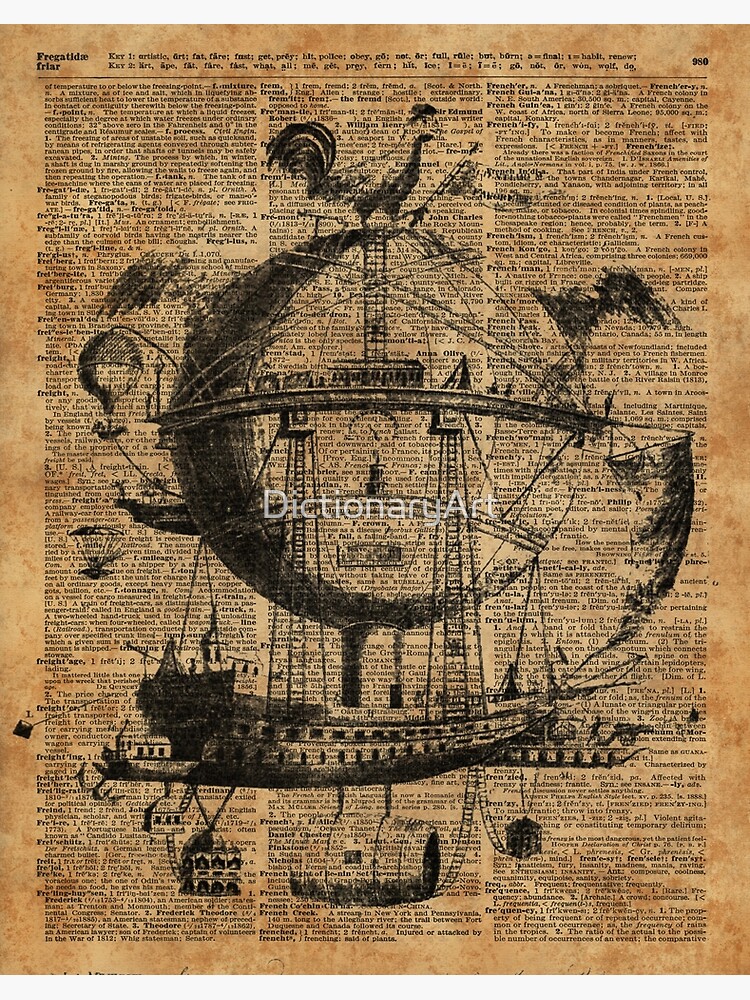The image depicts a fanciful, whimsical artwork superimposed onto an old, yellowed, and blotchy dictionary page. The paper itself is worn, with very small text arranged in three columns. There is a prominent white watermark in the center that reads "Dictionary Art," likely intended to deter image theft. The central figure in the artwork is an imaginative airship, combining elements of an old wooden ship attached to a large, round balloon encircled by a metal band. Atop the balloon stands a huge chicken or rooster holding a flag in its leg. 

Underneath the ship is a giant barrel, connected by rigging to ladders that extend from the bottom of the ship to various other elements. These include boxes and what appear to be small houses dangling from the ship, interconnected by additional ladders. The balloon itself features a structure resembling a meter or clock and has sails attached to the metal band around it. The rear of the ship features an anchor, and what seems to be a kite. 

In the background, other airships with different designs, such as one with a giant parachute, can be seen, further enriching the fantastical scene. The dictionary text beneath the artwork provides a textured backdrop, enhancing the vintage and surreal aesthetic of the piece.